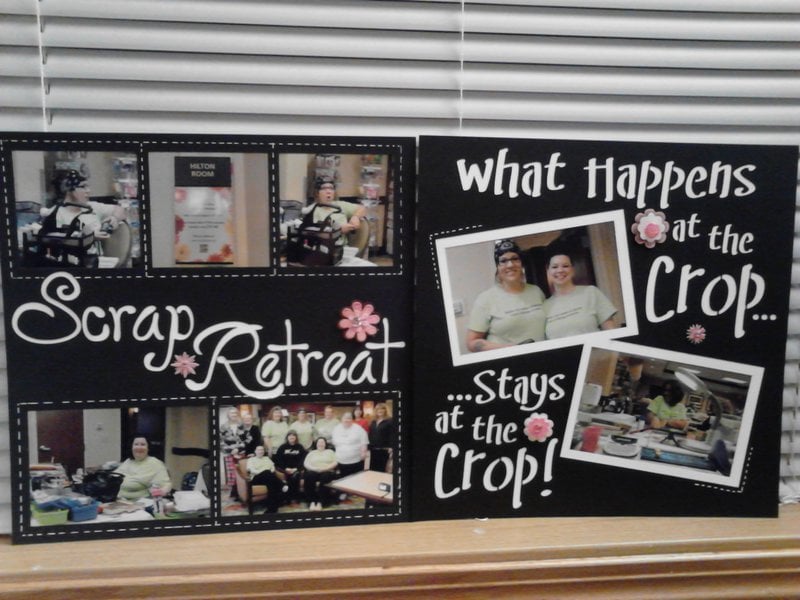This horizontal rectangular image depicts a meticulously crafted poster, showcasing a scrapbook-themed event. The scene is set indoors, possibly within a cozy home environment. The lower part of the image features a wooden, light tan-colored windowsill, while metallic blinds, currently closed, form the backdrop.

Centrally displayed on the windowsill, the poster is composed of two pages made from black rectangular paper. Each page is adorned with photographs and text interspersed with decorative pink flower stickers. On the left page, there are five photographs arranged with three at the top and two at the bottom, centered around white lettering that reads "Scrap Retreat." Delicate flower stickers embellish the area around the word "Retreat."

On the right page, a larger brown area hosts two photographs surrounded by white text that proclaims, "What Happens at the Crop Stays at the Crop." Pink flowers are also strategically placed around these images, enhancing the festive atmosphere suggested by the scrapbook. The overall color scheme includes hues of white, black, gray, orange, pink, and light green, contributing to the vibrant yet homey aesthetic of the poster.